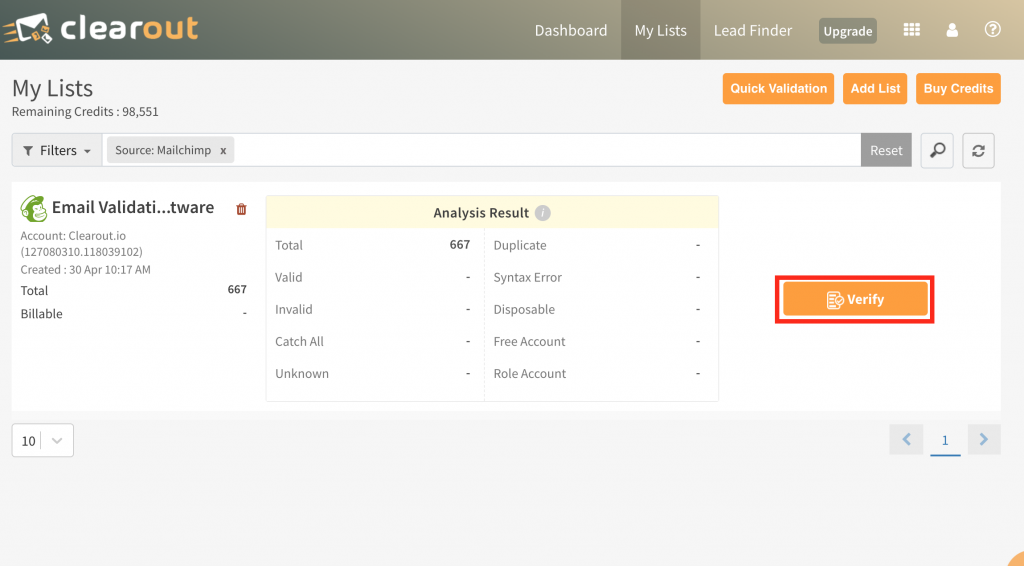This image displays the ClareOut website interface. The ClareOut logo is prominently positioned in the upper left corner of the screen. Adjacent to the logo on the top navigation bar, a menu is visible. On the far-right side of this bar, several navigation options are listed: "Dashboard," "My List," "Lead Finder," followed by an "Upgrade" button. 

The "My List" section is currently selected, as evidenced by the highlighted tab. This "My List" tab is not only marked on the menu bar but is also the focus of the main content area of the website. In the top-right quadrant of the main section, a summary box displays "Remaining Credits," which are listed as 98,551.

Below this, a lower section of the interface appears, offering email validation functionalities. Here, we see columns for account details and creation dates. To the immediate right of these details, an "Analyze Results" section is present. Adjacent to this, an orange "Verify" button with white text is positioned, providing users with the option to validate emails. The layout and color scheme clearly guide the user through the verification process, emphasizing functionality and ease of use.